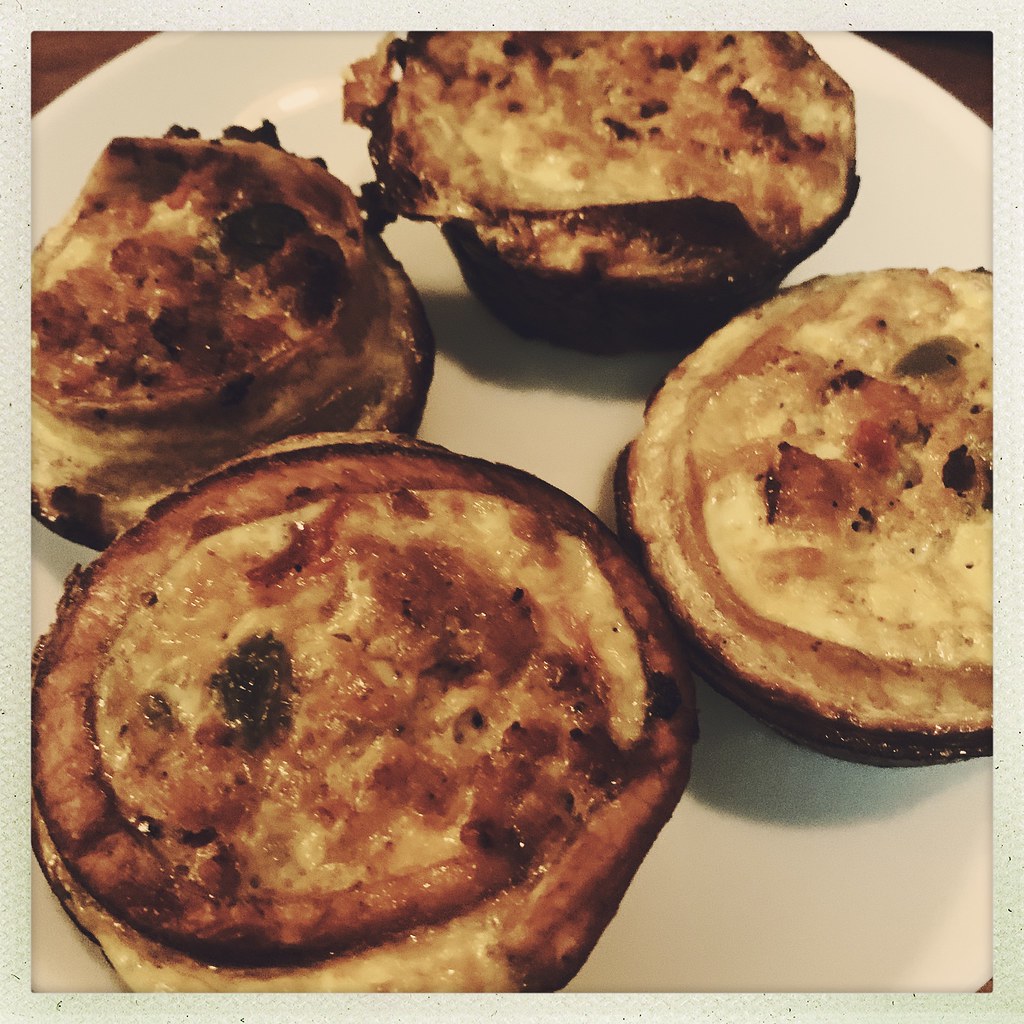The image is an artistic color photograph mounted on textured or watercolor paper, giving it a vintage, Polaroid-like appearance. It is a square photo taken from a slightly elevated angle, depicting four appetizing soufflés, which are positioned in a diamond pattern on a white plate. The top left corner of the image reveals a small portion of a brown background.

The warm, tungsten-colored lighting accentuates the soufflés' textures and colors, ranging from light yellow and light brown to dark brown and black. The tops of the soufflés appear crispy and browned, possibly topped with cheese that has broiled to a delectable finish. A few areas of the pastries look overdone, with some blackened portions indicating they were baked in cup-shaped depressions. This close-up photograph highlights the intricate details and shadowing of the food, suggesting a focus on the culinary appeal of the well-browned, cheesy soufflés.